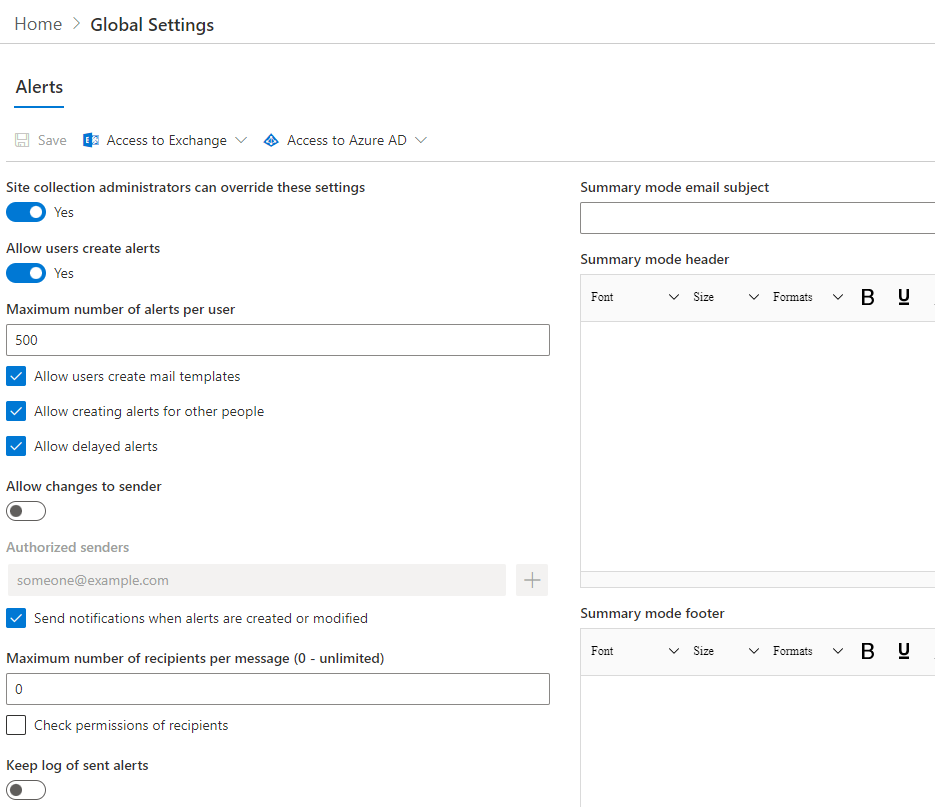**Caption:**

In the screenshot, various settings and options related to alerts and notifications within a web platform are displayed. At the top of the interface, accessible tabs include 'Home,' 'Global Settings,' 'Alerts,' 'Save,' 'Access to Exchange,' and 'Access to Store.' The highlighted configuration is for 'Site Collection Administrator Settings.'

Several toggle options allow users to tailor their notification preferences:
1. **Create Alerts:** Users can enable or disable the creation of alerts.
2. **Create Multiple Alerts:** Allows multiple alerts to be created per user.
3. **Allow Alerts for Others:** Grants permission to create alerts on behalf of other users.
4. **Delayed Alerts:** Enables or disables the sending of alerts after a specified delay.
5. **Change Notifications:** Allows or disallows changes that are not currently toggled.
6. **Authorized Sender:** Specifies that alerts must come from an individual at 'example.com.'

Additional configurations include:
- **Maximum Number of Alerts per User:** Set to 500.
- **Maximum Returns per Message:** Set to zero (unlimited).
- **Receipt Checking:** Options to monitor and confirm receipt of alerts.

Formatting settings include:
- **Font Size:** Specification defined.
- **Text Format:** Bold and Underline options are highlighted.

Rows of text reflect these configurations, emphasizing different user preferences and technical adjustments in a detailed, organized manner.